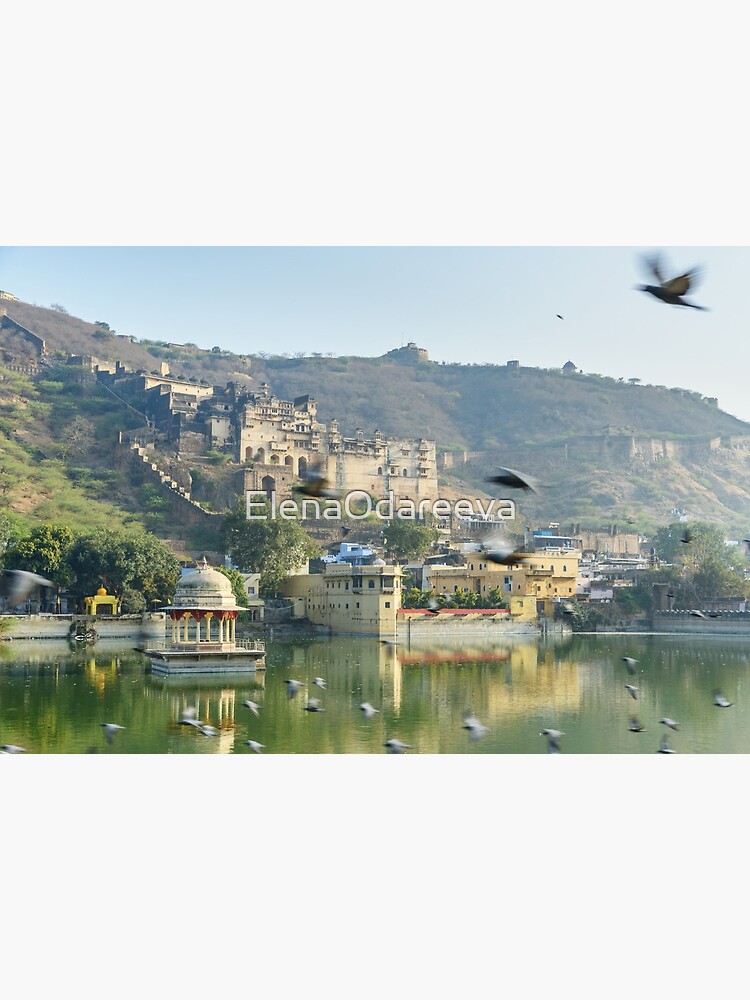This photograph, marked with a centrally located watermark reading "Elena Odariva," captures a serene seaside location, possibly in Asia. The composition divides into three major sections: the clear, calm green waters in the foreground, reflecting nearby foliage; a middle section featuring a few ivory and sand-colored buildings alongside retaining walls; and a steep, hilly terrain that dominates the background. Centrally situated on the hill is a castle-like structure, adding an element of grandeur to the scene. The bright, clear blue sky suggests sunny, perhaps early morning weather. The image is animated by numerous birds in flight, ranging from larger ones in the upper right corner to smaller ones scattered lower, all appearing slightly blurry due to their motion. Notably, a gazebo-like structure with an onion-shaped top rests on a man-made island within the calm lake, adding cultural intrigue to the picturesque landscape.